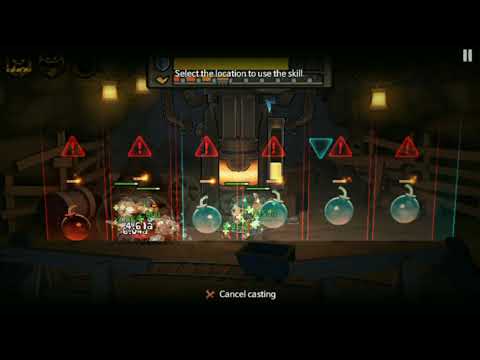The animated image appears to be from a video game and features a dark, mine shaft setting with yellow lanterns hanging from the ceiling, illuminating the surroundings. At the heart of the image is a line of six cartoon-styled bombs, arranged horizontally and roughly centered. The first two bombs from the left are red, with the second partially obscured by small text and brown symbols, likely indicating it's in the process of exploding. The remaining four bombs are blue, each with red caution symbols inside red triangles hovering above them. The bombs resemble round glass jars with either stems or fuses on top. 

At the top of the image, white text reads "Select the location to use the skill," indicating an interactive game element. Near the bottom, a black mine cart rests on gray mine tracks, with the words "Cancel casting" in white text accompanied by a red X icon to its left. The edges of the image are notably dark, with some reflections suggesting possible character presence. The overall scene suggests a moment of imminent action or decision within a gameplay context, enhanced by a pause button located at the top right.